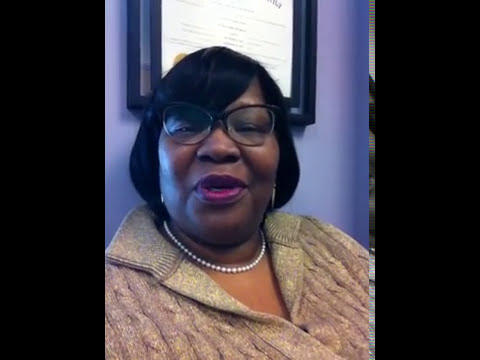The image features a close-up portrait of a middle-aged African-American woman with dark black hair, parted to the left and hanging down to around shoulder length. She is wearing round, black-framed glasses and has pink-purple lipstick enhancing her wide, smiling face. She is adorned with a pearl necklace and a light gray, textured cardigan that features a ribbed pattern and a large collar. Her body is angled slightly to the right while she looks directly at the camera. The background consists of a light purple wall, and there's a black-framed diploma or certificate directly above her head, suggesting she might be in an office setting. The sides of the image have black rectangular bars, emphasizing the central focus on the woman.